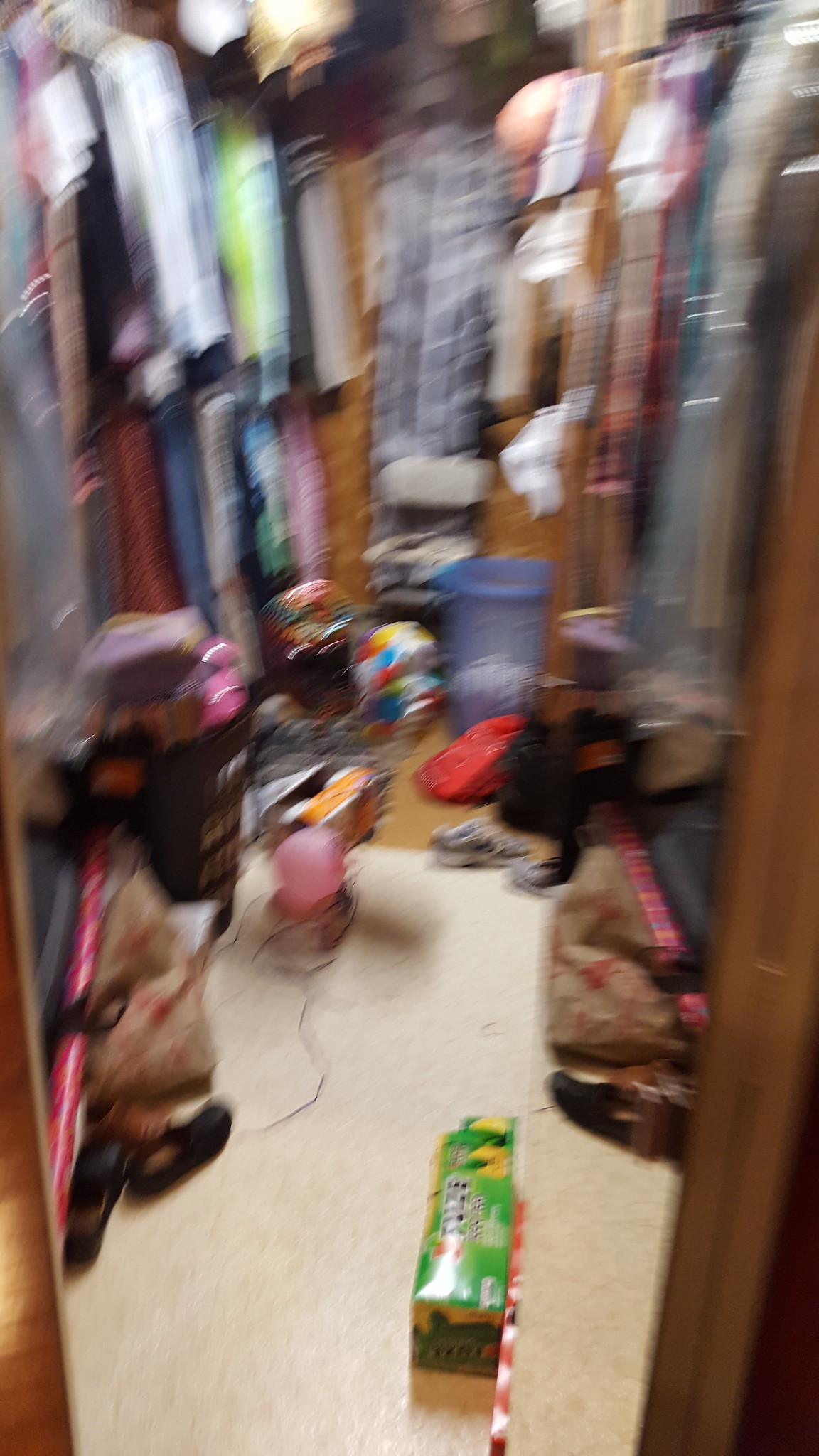The image depicts the interior of a closet with a slightly blurry focus. The floor is covered in a light beige carpet, suggesting a soft and neutral base. The closet door is made of brown wood, adding a warm, earthy tone to the scene. In the back, a blue dress adorned with floral patterns is hanging, providing a splash of color and charm. A small blue trash can is visible, positioned unobtrusively. At the front of the closet, a green-topped box with red and white stripes along the side adds a hint of eclectic organization. The closet offers ample hanging space, though it is currently filled with various items. On the floor, there are scattered clothes, including some neatly folded pants situated to the right. Among the clutter, a bottle containing pink liquid stands out, adding curiosity to the assortment of objects. Overall, the closet displays a combination of utility and disarray, filled with everyday items and personal belongings.